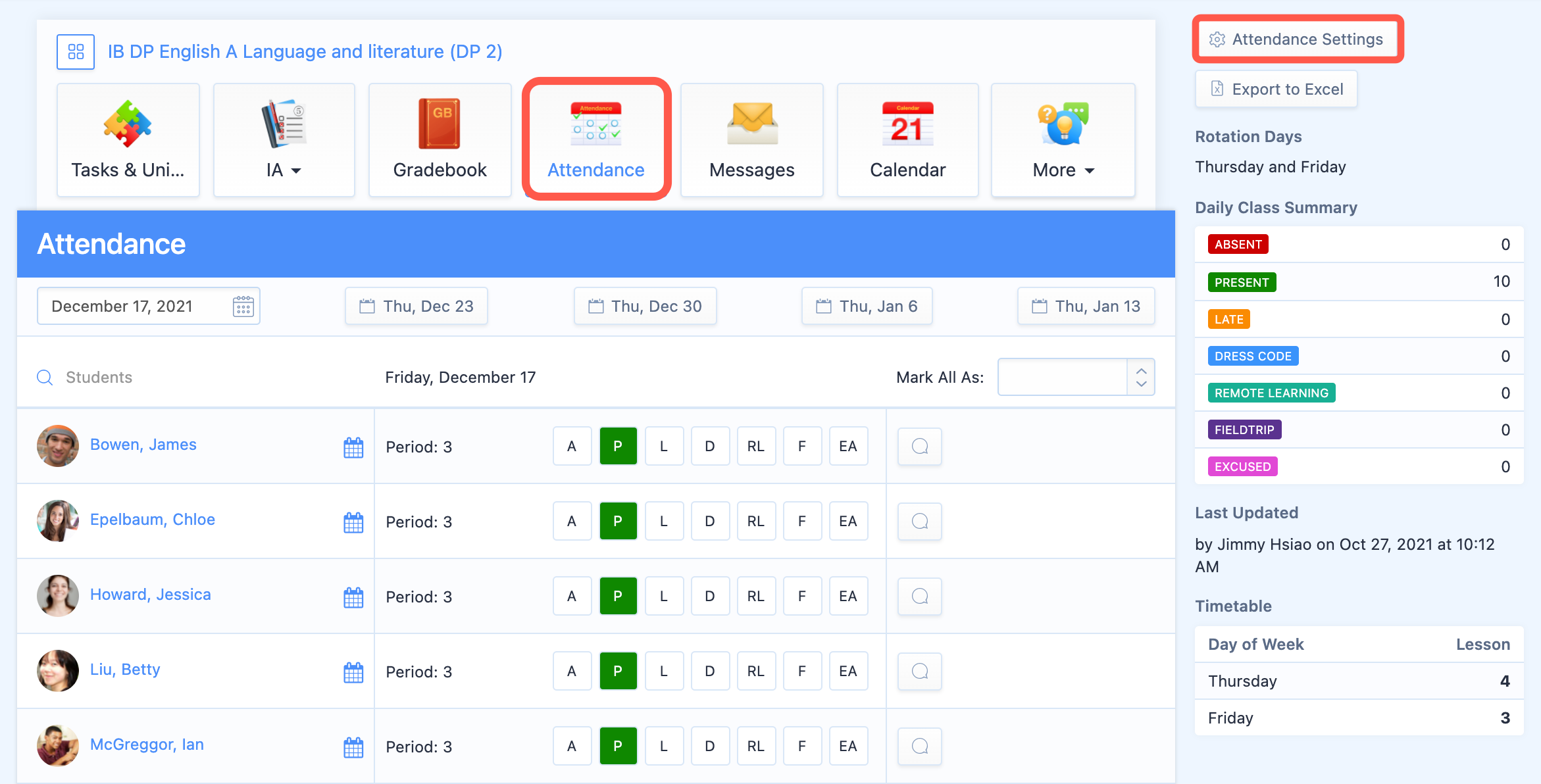The vibrant webpage of an academic portal displays a multitude of colorful elements against a predominantly white background. At the top, the heading reads "IB DP English A: Language and Literature DP2" in bold blue letters. The webpage is adorned with a variety of colors: white, blue, red, purple, green, dark purple, and orange.

Several icons are visible, including tasks and university-related symbols. Colorful puzzle pieces in green, blue, red, and yellow are seen, possibly representing different categories or sections. The IA section features a dropdown menu for additional options. A piece of paper icon accompanies a pencil, symbolizing note-taking or assignments.

The gradebook is represented by an orange book icon with "GB" inscribed on it. Attendance, which has been highlighted in red, is also prominently listed in blue and is associated with a calendar icon featuring red, white, and blue colors. Next to the "Messages" section, there's an envelope icon, while the calendar option is marked with a red and white calendar icon.

A "More" dropdown menu provides further functionalities. To the right side, the attendance and settings icons are highlighted in red, drawing attention to these important features. An "Export to Excel" option is available, likely for data export purposes. The rotation days for Thursday and Friday are indicated in blue.

The daily class summary section shows a white square divided into colorful segments. Here, "Absent" is marked with zero in red, "Present" is highlighted with 10 in green, "Late" is zero in orange, and "Dress Code" compliance is zero in blue. 

Overall, the webpage is a detailed, user-friendly interface designed to organize and present educational information efficiently.